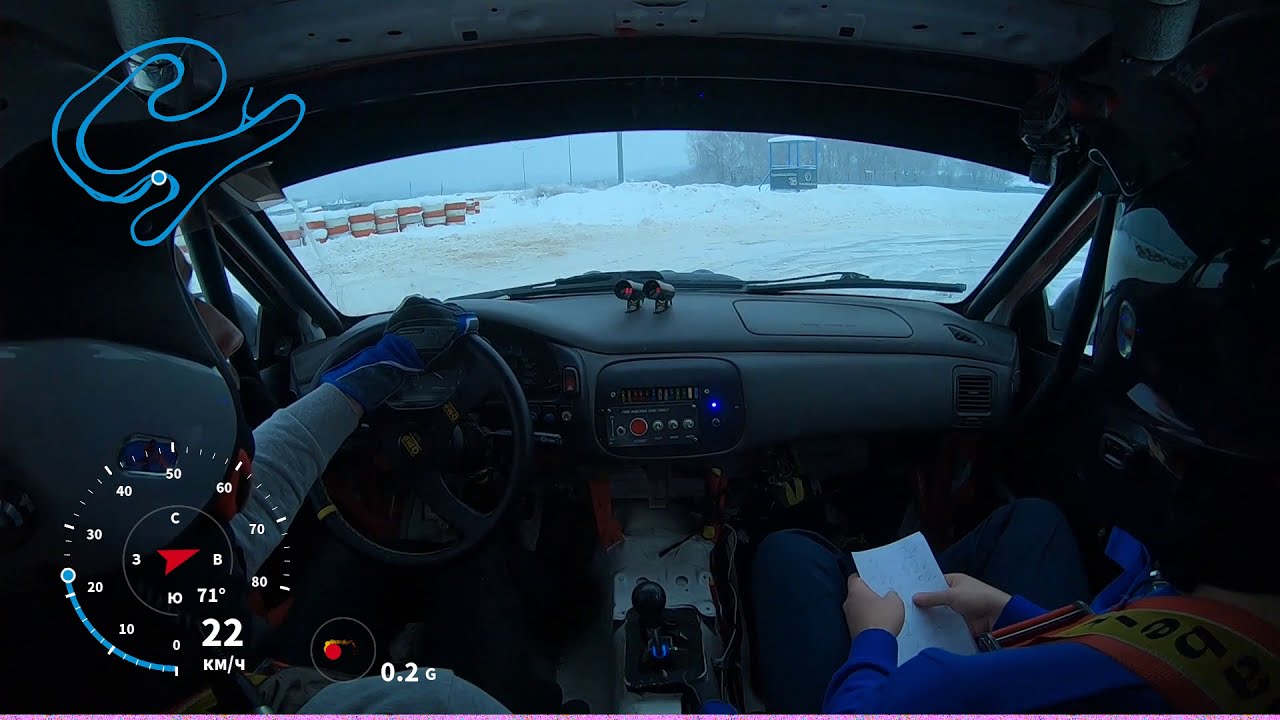Inside the vehicle, the driver on the left, dressed in a gray sweatshirt and a black and gray helmet, is gripping the steering wheel with a dark blue and black gloved hand. The passenger on the right, also wearing a helmet and secured with racing straps, dons a blue jacket and blue jeans, holding a white piece of paper with indistinct writing. The car's dashboard displays a digital track map in the upper left corner, showing their current position as a blue dot on a blue track. Below this display, the speedometer reads 22KM/4 with a 0.2G notation, indicating a speed around 22 km/h. Outside the windshield, a slow-moving lane stretches ahead, bordered on the left by numerous white buckets with red lines, and on the right by a booth with a green bottom, black midsection, and white top. Directly ahead lies a circular pole surrounded by trees.